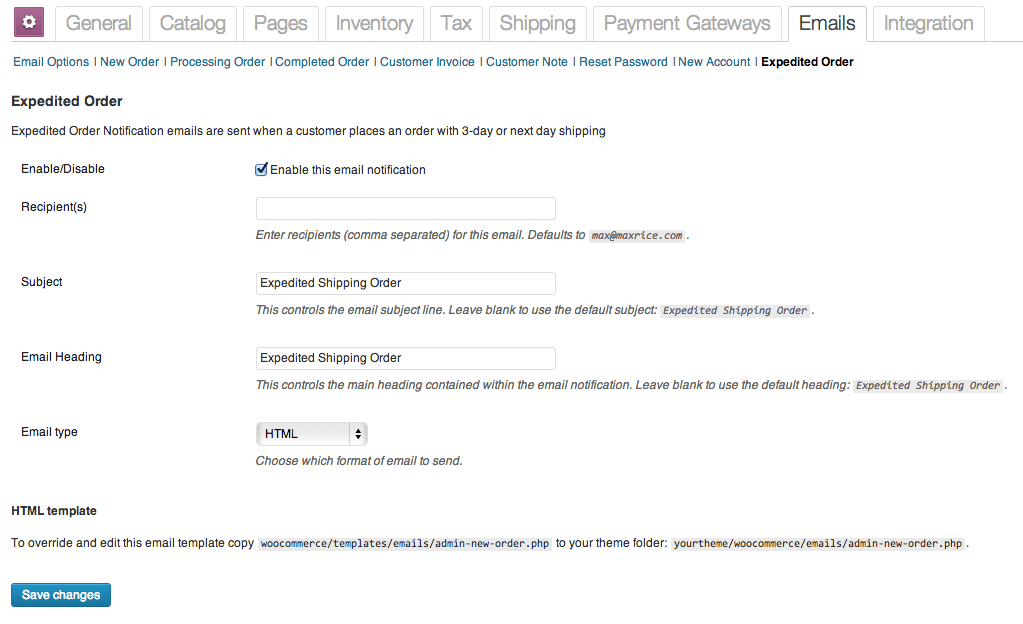This is a detailed screenshot of the "Emails" settings page on a particular website. The interface features multiple tabs at the top, starting with a purple square containing a settings gear icon. The visible tabs in order are: General, Catalog, Pages, Inventory, Tax, Shipping, Payment Gateways, Emails (which is currently highlighted), and Integration. 

Under the "Emails" tab, there is an extensive list of categories available for configuration:

1. **Email Options**
2. **New Order**
3. **Processing Order**
4. **Completed Order**
5. **Customer Invoice**
6. **Customer Note**
7. **Reset Password**
8. **New Account**
9. **Expedited Order** (highlighted)

Below the highlighted "Expedited Order" category, the heading "Expedited Order" is in bold black font. The accompanying text explains that expedited order notification emails are sent when a customer selects three-day or next-day shipping options.

The settings options for "Expedited Order" are as follows:

- **Enable/Disable**: The option to enable this email notification is highlighted with a checkmark.
- **Recipients**: There is an empty text box for entering recipient email addresses, separated by commas. 
- **Subject**: The text box labeled "Expedited Shipping Order" controls the email subject line.
- **Email Heading**: The text box contains the heading "Expedited Shipping Order," which controls the main heading of the email.
- **Email Type**: A dropdown menu with arrows for scrolling up and down; HTML is highlighted, indicating the chosen email format.

There is a heading for "HTML Template" which suggests that to override and edit the email template, one must copy the provided webpage into their theme folder.

At the very bottom of the screen, there is a blue bar labeled "Save Changes" for saving any modifications made to the settings.